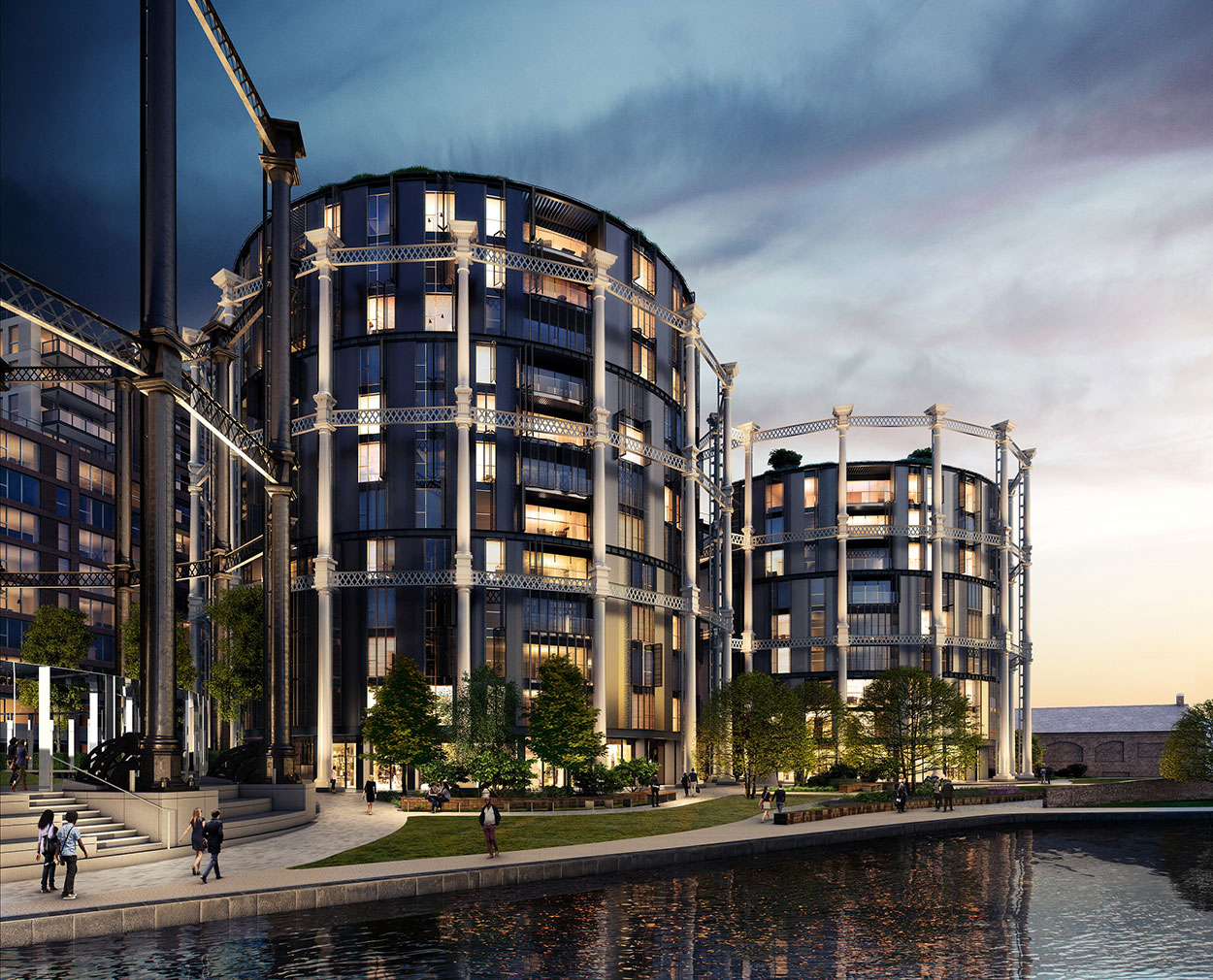This detailed image appears to be an outdoor waterfront scene, potentially AI-generated or an actual photograph. The foreground features a lake extending from the bottom right-hand area, narrowing as it stretches towards the left. This body of water may resemble a canal, comparable to those found in Venice. On the opposite bank, sidewalks and grassy areas create a path leading to three distinctive buildings. These structures include two large, round, multi-storied buildings and one rectangular one. 

The buildings, rising approximately ten stories high, are impressive with their modern appearance. Surrounding them is a scaffolding-like structure, reminiscent of artistic cages rather than traditional support columns. This decorative scaffolding encapsulates the buildings, adding an intricate aesthetic layer. Many windows in these high-rises are lit, contributing to the lively atmosphere of the scene.

In the distance, a footbridge can be seen, potentially leading pedestrians across the canal. The sky forms a backdrop transitioning from light white at the horizon to dark blue towards the top left corner, enhancing the visual depth. Additionally, scattered individuals in modern attire stroll along the lake's perimeter, adding a human element to the serene, yet urban, landscape. The water itself presents a mix of black and blue hues, reflecting its surroundings elegantly.